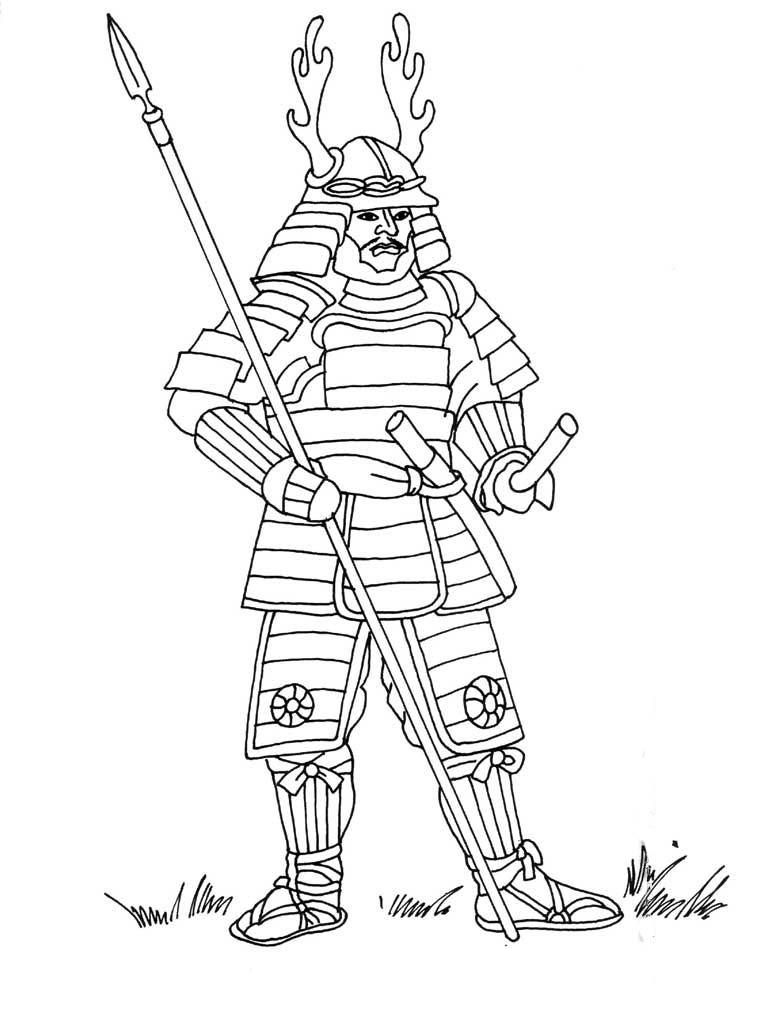The image depicts a detailed black and white line drawing, reminiscent of something you might find in a coloring book or a sketch. At the center stands a samurai warrior adorned in full body armor. The samurai's helmet is intricately designed with ribs running along the sides and is topped with antler-like horns, giving it a distinctive appearance. The helmet also features a chain circling around the top. He exudes seriousness with his stern facial expression and visible facial hair.

In one hand, the samurai grips a long spear with a sharp tip, extending upward past his head. His other hand holds what appears to be a sword, sheathed at his belt. He also wears strapped sandals, and around his knees, there are circular designs on his armor. The samurai stands firmly in a small field of grass set against a plain white background, further emphasizing the focus on the warrior. The absence of text and the monochrome palette suggest a simple yet striking artistic print or poster.